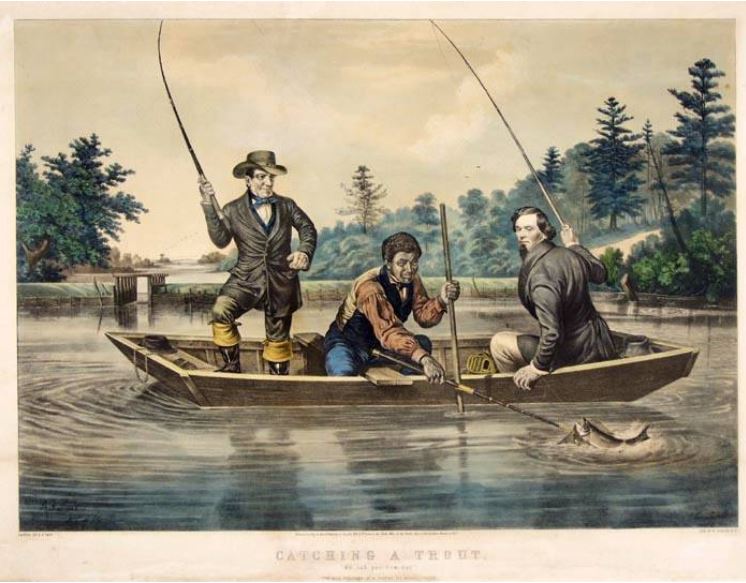The painting titled "Catching a Trout" depicts a scene reminiscent of colonial or pre-Civil War times, featuring three men in a wooden boat engaged in fishing on a serene lake or pond. Dominating the left side, a man stands confidently in black pants, black and yellow boots, an overcoat, and a cowboy hat. He holds a fishing rod mid-action. In the middle of the boat, another man, dressed in a black and brown upper garment and blue pants, sits on a wooden plank. He uses one hand to grip a net while his other hand holds a fishing rod, successfully trapping a trout. The third man sits on the right with his back partially turned towards the viewer, wearing a grey jacket and off-white trousers. He has long hair, a goatee, and is partly turned to observe the catch, holding the boat steady with one hand and a fishing rod with the other. The background is filled with lush trees and hints of mountains under a sky that transitions into a bright yellow tint, evoking a sense of calm. The water surrounding them ripples gently, adding to the realism of the scene. The painting is bordered by a peach-colored frame, with the title "Catching a Trout" inscribed at the bottom in gray font.